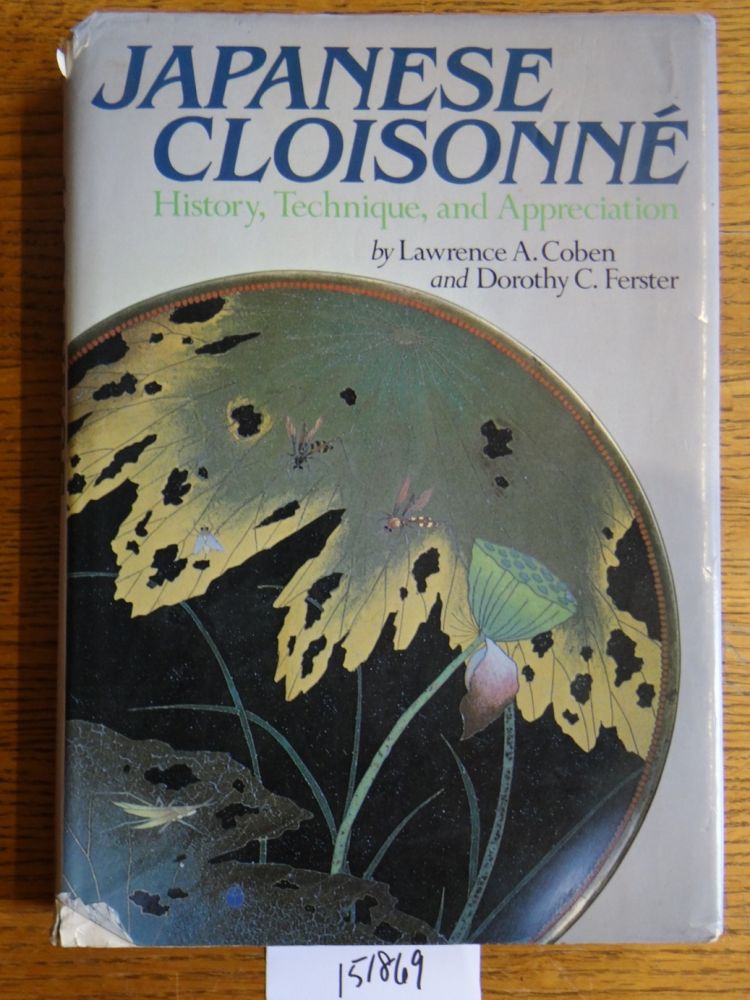The photograph showcases a detailed, vertically rectangular, full-color image captured indoors under artificial lighting. Dominating the scene is a hardcover book, delicately placed on a mid-range brown wooden table, with clearly visible wood grain patterns. A small strip of paper with the handwritten number "151869" lies at the lower center of the image. The book's white protective cover features the title "Japanese Cloisonné" in bold blue letters, followed by the subtitle "History, Technique, and Appreciation" in green. Authored by Lawrence A. Cohen and Dorothy C. Furster, as indicated in black text, the cover is adorned with a detailed illustration of a bluish spherical object. This sphere, bordered in silver-brown, displays a rich, night-sky-like background adorned with a collection of intricately drawn, tattered leaves in shades of yellow, green, and dark gray, accompanied by various insects including crickets and honeybees. Additionally, a small flower with green and pink hues adds to the intricate design, which appears to be cartoonishly magnified, enriching the cover with a vivid and complex visual narrative.